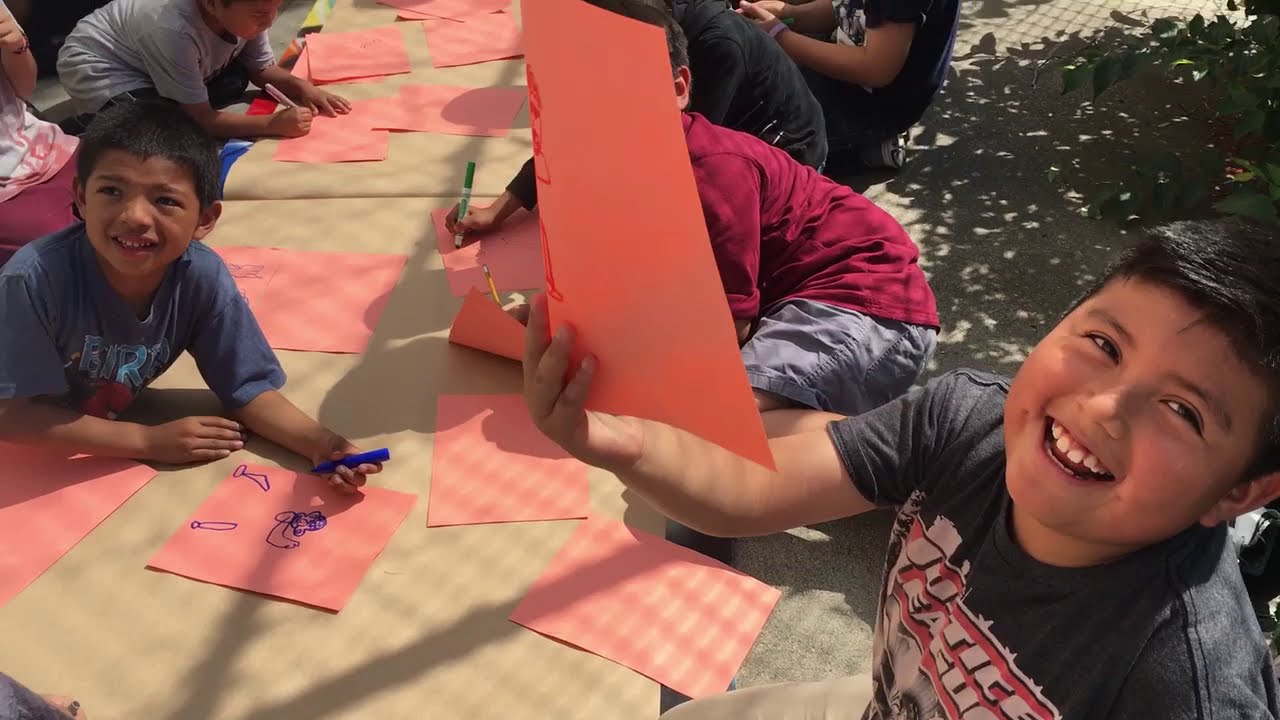The photograph features a group of children engaging in an outdoor activity, likely related to school or a special event. They appear to be around eight or nine years old, predominantly boys, all sporting short hair and dressed in t-shirts and shorts. The setting is bright and sunny, and the kids are either seated on the ground or at a brown-paper-covered table, possibly to protect the surface. They are drawing on salmon-colored pieces of paper with various writing tools, predominantly blue and green markers, although pencils are also evident. Several pieces of these papers are scattered around as they enthusiastically work on their creative projects. A child in the foreground on the left is notably focused, doodling with a blue marker, while another in the foreground on the right is smiling brightly and seems to be handing his paper to someone out of frame. The general atmosphere is joyful and engaging, with many children displaying happy expressions as they participate in this arts-and-crafts activity.